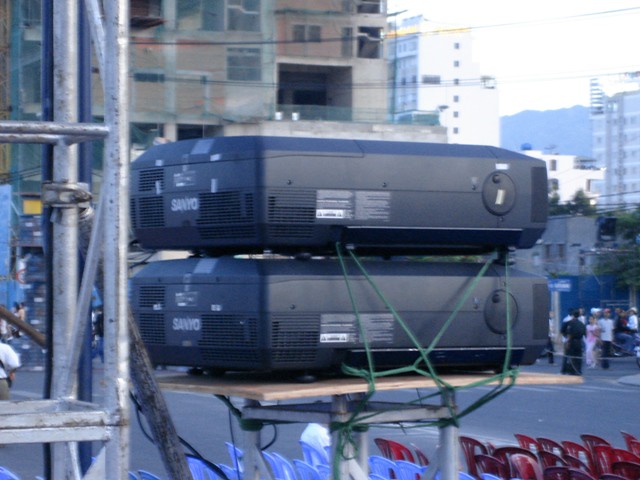This is a color photograph taken outdoors in an urban area, capturing a somewhat blurry scene on a city street. The focal point of the image is two rectangular electronic devices, possibly projectors, stacked on top of each other. These devices, black in color and marked with the word "Sanrio" in white, are mounted on a narrow wooden pedestal. The pedestal is supported by a structure comprising metal bars with four legs. Green cords can be seen connecting and securing the devices to the mount. Each device has vents on the sides and circular elements on the right. In the background, a cityscape of tall greyish and brown buildings is visible under a white sky. On the left side of the image, there is chrome-colored iron scaffolding. To the right, there are blurred figures of people and several rows of plastic chairs in red and blue hues. The scene suggests a public event or meeting, possibly utilizing the devices for display or projection purposes.